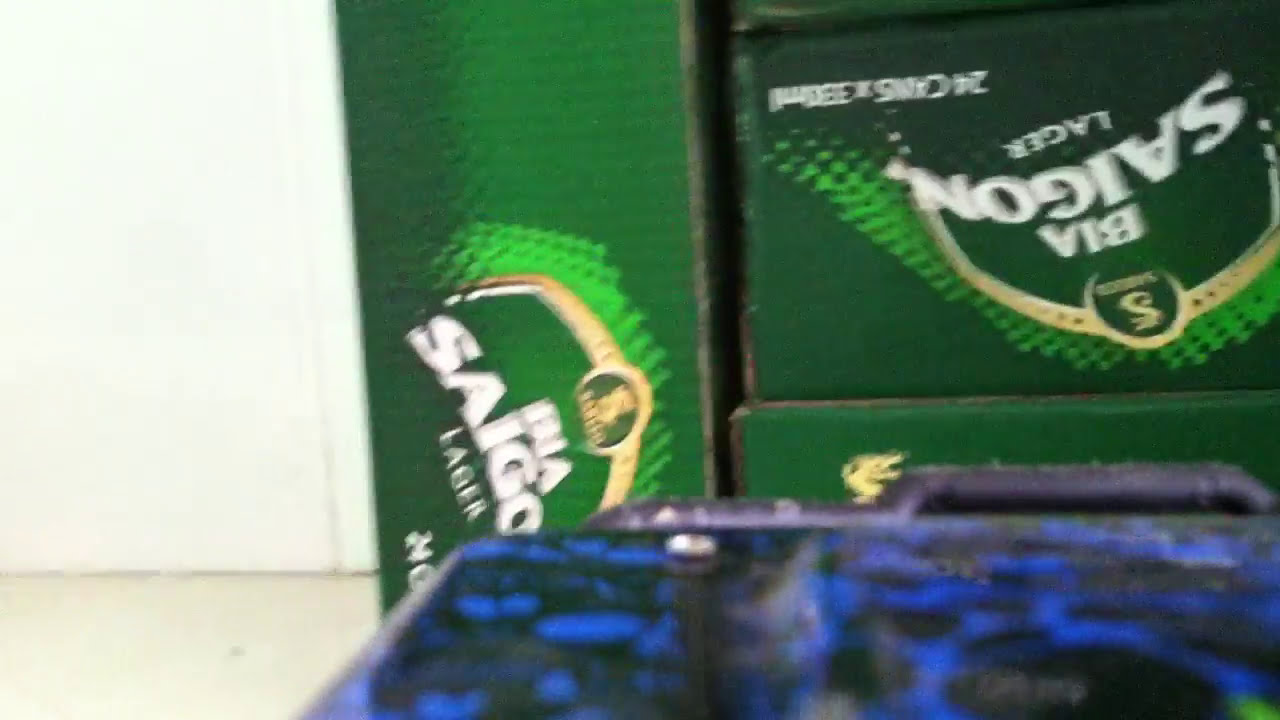This blurry image features a stack of green cardboard beer boxes with gold accents and white lettering. Each box prominently displays "BIA SAIGON LAGER" in bold, white, all-caps letters, with the word "Saigon" angled and "24 cans" written horizontally below it. The boxes are arranged with one turned on its side, another upside down on top of an upright box, forming a small tower of three. Above the gold decoration, you can see some light green shading. To the front and bottom right of the boxes, there appears to be a blue and black object, likely a suitcase or briefcase, identifiable by its flat top and black handle. The background includes a white wall and an off-white floor, with a dividing line suggesting a counter or lower wall section on the left side of the image.